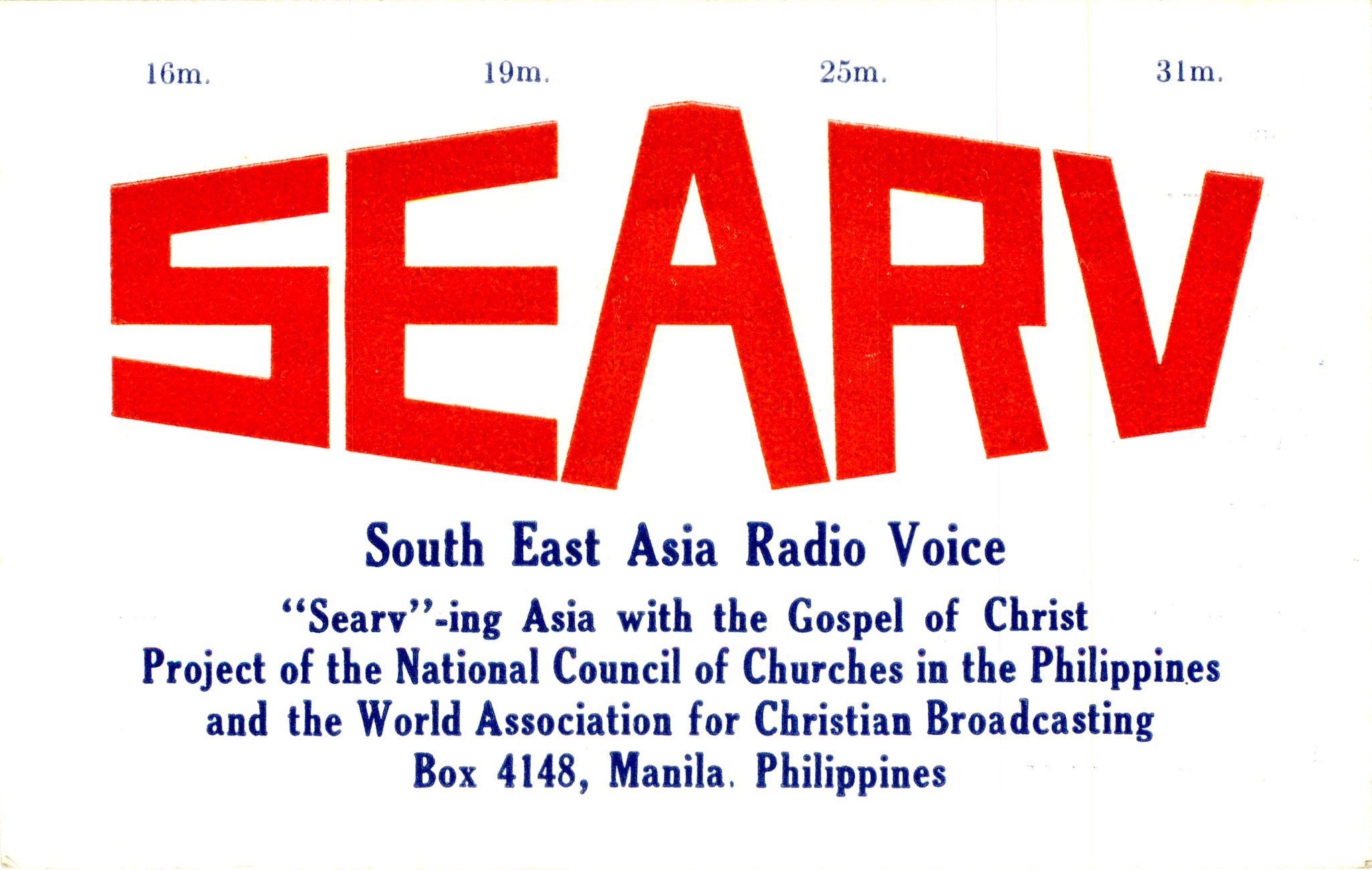The image features a rectangular white background with multiple lines of text. In the upper left corner, small blue text reads "16M, 19M, 25M, 31M." Dominating the center, large bold red letters spell out "SCARV" in a distinctive font where the 'A' arches uniquely. Beneath this, much smaller blue text includes "Southeast Asia Radio Voice, Serving Asia with the Gospel of Christ, Project of the National Council of Churches in the Philippines and the World Association for Christian Broadcasting." Additionally, the address "Box 4148, Manila, Philippines" is specified. The corners of the card exhibit small marks, suggesting it may have previously been tacked up, perhaps indicating its use as a promotional banner for the radio station.